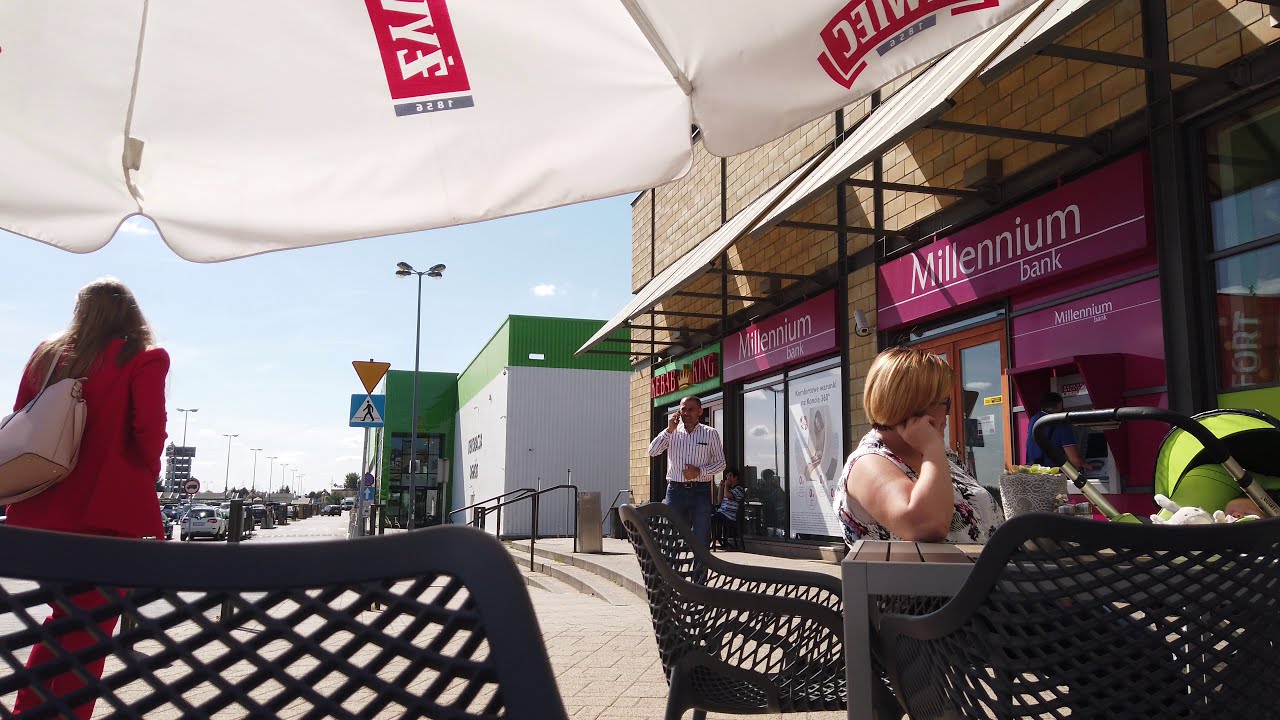The image is a casually taken, landscape-oriented color photograph of an outdoor restaurant setting along a city sidewalk, capturing a scene filled with lively colors and intricate details. In the foreground, tables with black woven chairs, characterized by a grid pattern that allows visibility through the backings, are positioned under white umbrellas with red lettering. To the left, a woman in a striking red pantsuit, carrying a large beige pocketbook, walks away from the viewer on the cobblestoned path. On the right side of the image, a woman with short blonde hair and sunglasses sits at a gray table, dressed in a sleeveless shirt. Next to her, a baby in a stroller is visible, with just the top of the baby's head peeking out. Above and slightly behind her, a sign reading "Millennium Bank" in white letters on a purple background is affixed to a brown brick building with a canopy. Further to the background, parked cars, lampposts, storefronts, and pedestrian crossing signs are visible, adding depth to the bustling street scene. A man is seen talking on a phone while walking along the sidewalk. The photograph vividly captures the local ambiance, blending the immediate interactions with the broader cityscape.